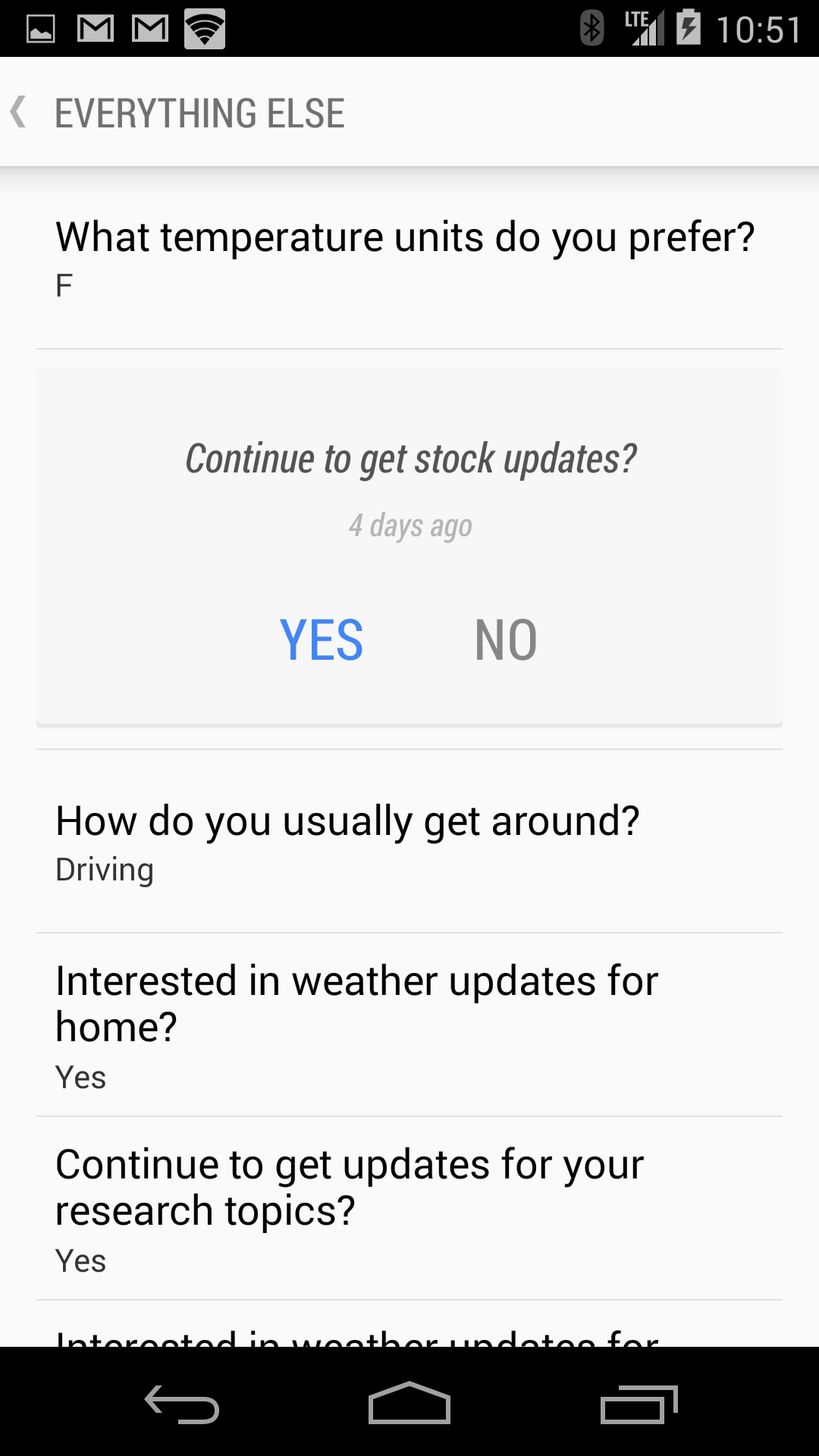The image captures a smartphone screen displaying a settings or preferences page from an application. The top of the page is titled "Everything Else," followed by a section asking, "What temperature units do you prefer?" with a lowercase "f" next to it, indicating the option for Fahrenheit. Below, a faint gray line separates this section from the next query that reads, "Continue to get stock updates?" This is followed by a timestamp that says "four days ago," and two choice buttons - "Yes" in bold blueprint and "No" in gray print.

The subsequent section inquires, "How do you usually get around?" with the option "Driving" chosen. Next, it asks, "Interested in weather updates for home?" answered with "Yes." This is followed by a prompt, "Continue to get updates for your research topics?" also answered with "Yes."

Further down, another question begins with "Interested in weather updates for," but the rest of the text is truncated by a black rectangle at the bottom of the page. This black rectangle contains three icons: a refresh arrow, an envelope symbol, and an overlapping rectangle icon, resembling a documents or tabs symbol.